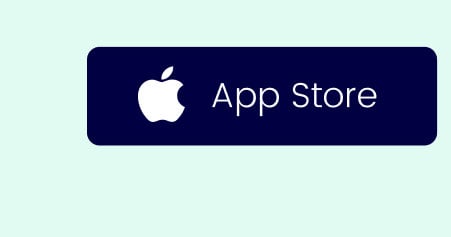The image features a "Download on the App Store" button prominently placed against a light mint-colored background. The button, approximately in the lower right quadrant of the image, is slightly off-center to the right and positioned about 60% down the page. The background beneath the button extends further compared to the top, perfectly accommodating the button's height. The button itself is a dark hue, appearing either in black or deep blue. Its edges are rounded, adding a sleek look to its design. Central to the button's design is the white text that reads "App Store." To the left of this text is the iconic Apple logo, also in white, featuring an apple with a distinctive bite taken out of its right side and a leaf slanting to the right. The overall composition is minimalist, ensuring the button remains the focal point.